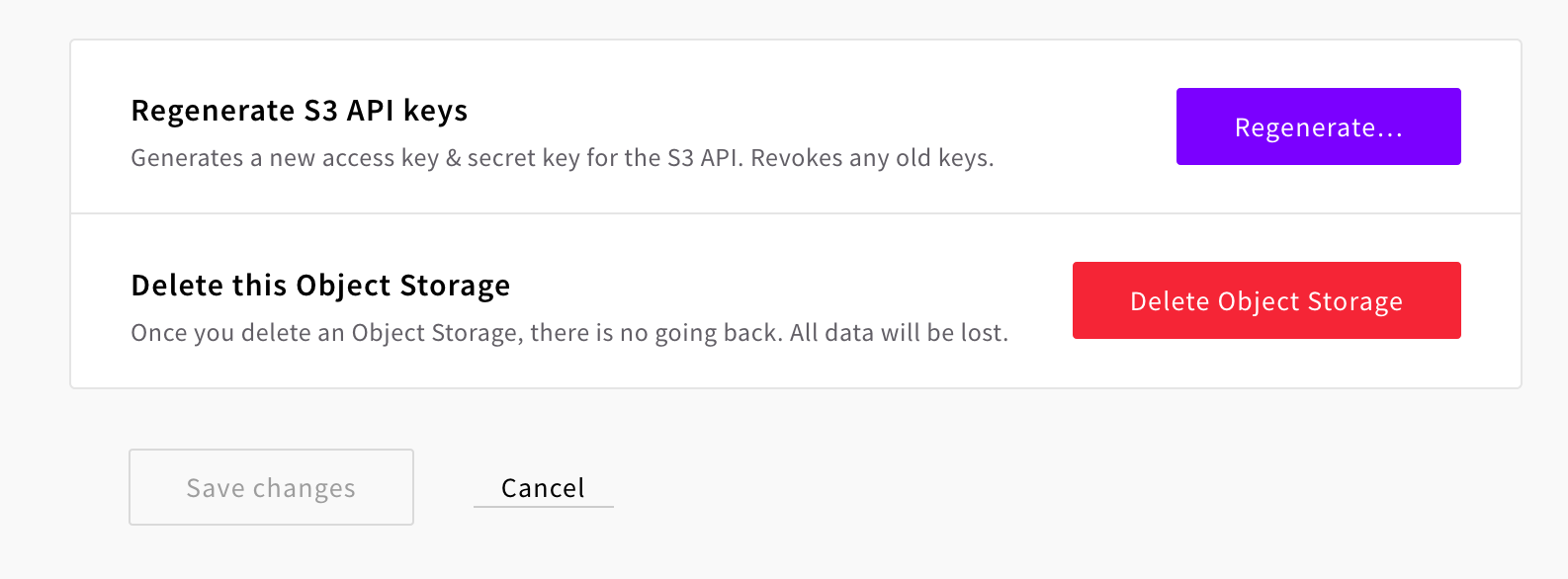Screenshot Description:

The screenshot displays a simple interface featuring two dialogue boxes within a larger gray rectangular dialogue box. 

The first dialogue box, prominently positioned at the top, is designed to manage API keys. It includes a clear, bold title: "Regenerate S3 API keys." Beneath this title, a brief explanation informs the user that selecting this option will generate new access and secret keys for the S3 API, while revoking any old keys. Adjacent to this explanatory text is a prominent purple button labeled "Regenerate..."

Directly below this, the second dialogue box provides an option for data management, titled in bold: "Delete this object storage." The accompanying subtext warns the user that this action is irreversible and will result in the loss of all data. This section features a striking red button labeled "Delete Object Storage."

Neither option appears to have been selected, as indicated by the inactive (grayed-out) "Save Changes" button at the bottom of the interface. This suggests that the user has not yet made any changes or decisions concerning the available options. The "Cancel" button is positioned nearby, providing an alternative to undo or exit the dialogue.